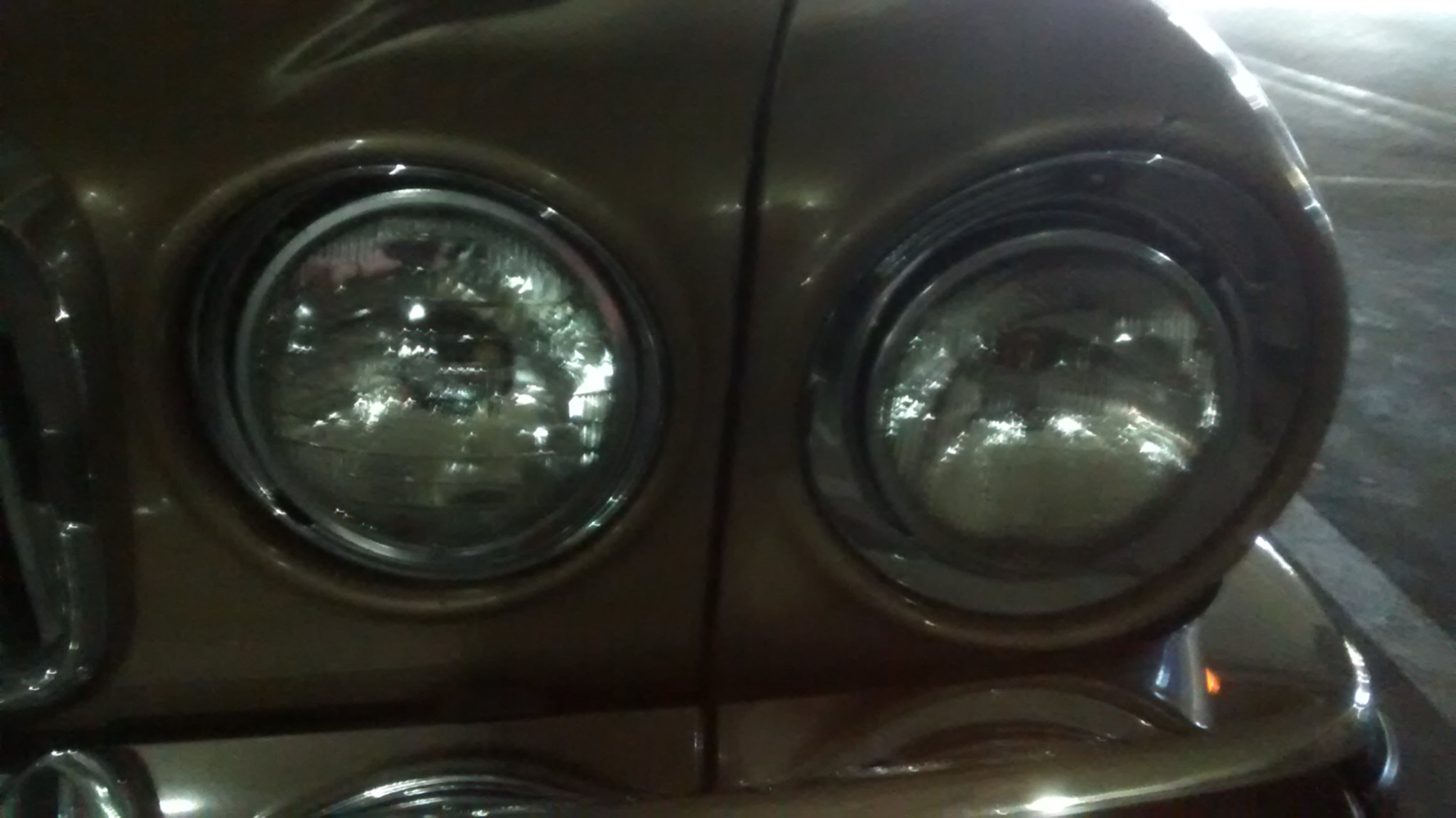This image is a blurry, close-up photo of part of an old automobile, captured at a 45-degree angle. The vehicle appears to be gold or silver in color, though the image is so dull and dark that it's hard to be certain. The main focus is on two round, clear headlight lenses, positioned next to each other with the right light housed in a curved casing on the outer edge of the car. Below the headlights, a curved bumper or fender is visible, suggestive of a 1960s or early 70s vehicle, highlighted by chrome plating beneath the lights. To the left of the headlights, a portion of the grille is visible. In the background on the right side of the image, there's black asphalt with a white line, a travel lane marked by a double yellow line, and part of another lane, indicating the car is parked in a parking lot. The overall image is quite dull and blurry, with reflections in the headlight lenses but no clear details, capturing a scene that feels almost panoramic.